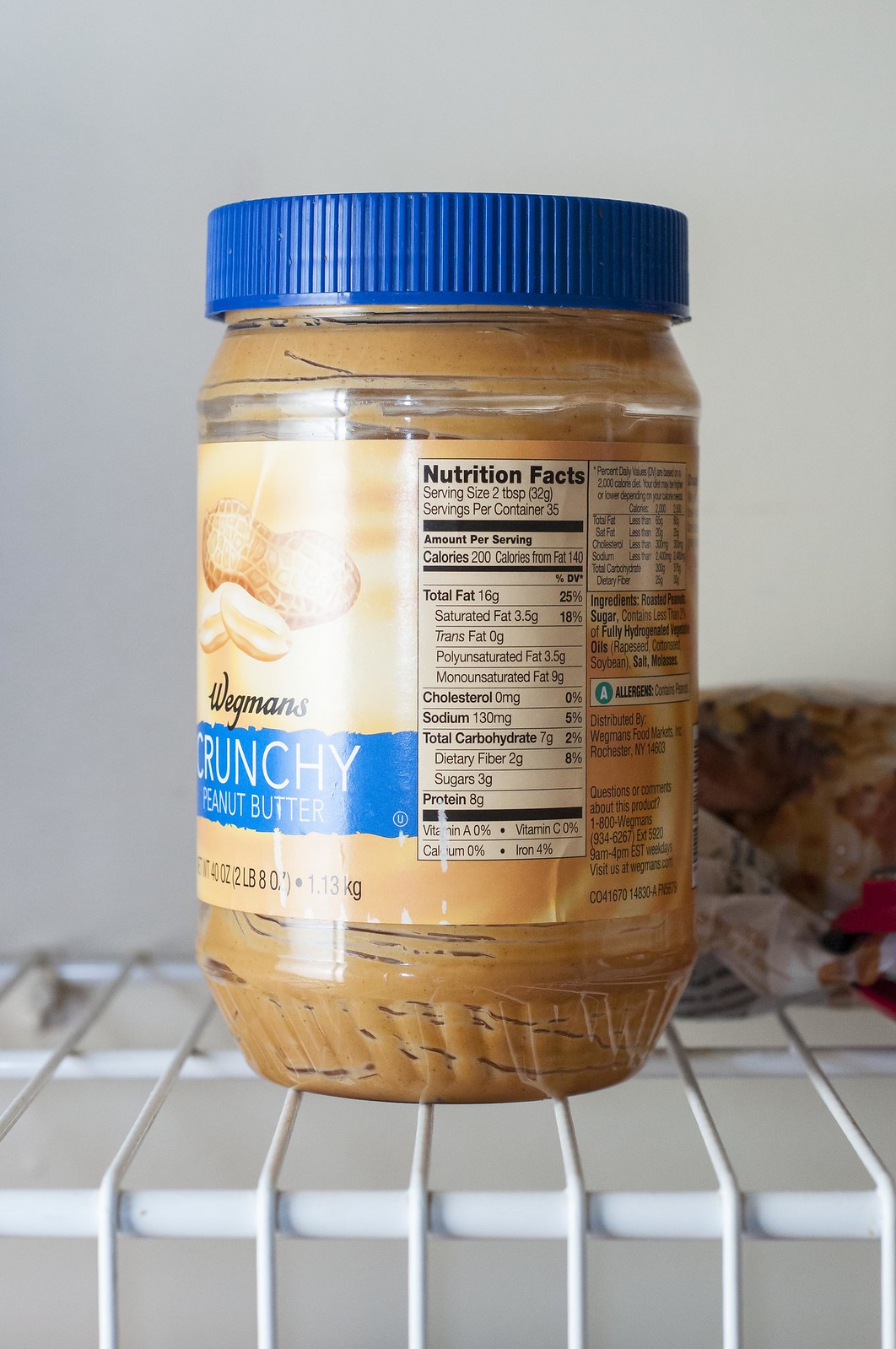This vertical, rectangular color photograph captures a nearly empty jar of Wegmans Crunchy Peanut Butter, placed on a white, plastic-coated wire shelf, possibly inside a refrigerator. The clear glass jar, which reveals remnants of peanut butter along its sides, features a beige label adorned with pictures of peanuts—both in-shell and shelled—at the top. The brand name "Wegmans" is prominently written in black script on the label. Below it, a bright blue strip displays "CRUNCHY PEANUT BUTTER" in white letters. Further down, the jar's weight is indicated as "2 pounds 8 ounces (1.13 kilograms)" in dark brown text. The label also shows the Nutrition Facts box in dark brown text on an off-white background, listing typical nutritional information per serving, including calories, fats, proteins, and vitamins. To the right of the Nutrition Facts, there's additional product information, including distribution details by Wegmans Food Market, Rochester, New York, and a customer service contact number. In the background, a greenish plastic bag containing brown and green items is partially visible.